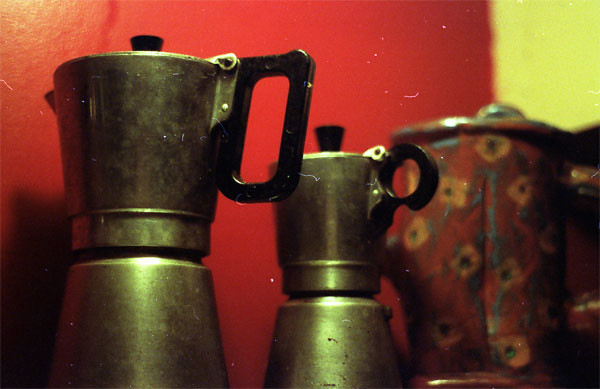The image is an indoor, color close-up of two vintage espresso coffee makers positioned side-by-side to the left of the frame. Both espresso makers feature a tarnished tin construction with a black plastic handle extending upward and a small black knob on top of the metal lid. The one on the left is slightly larger and closer to the camera than the one on the right. Positioned to the far right of the image is a larger ceramic container, distinguished by its red color adorned with floral designs. The background is dominated by a red wall, with a hint of bright yellow in the upper right corner. The image has a slight blur in the background, emphasizing the aging coffee makers in the foreground.